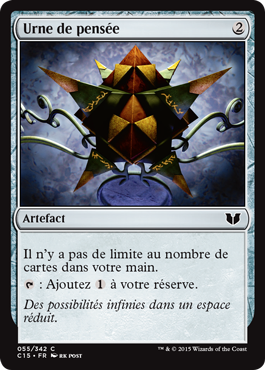The image depicts what appears to be a collectible card similar to a Pokémon card, characterized by a vertical rectangular shape with rounded corners. The card's design begins with a black border framing the entire card. Inside this black border is a slightly smaller border in a light blue color, adorned with various black and white specks.

At the top center of the card, there is a silver oval shape, with black text situated at the top left that reads "Earned it Pensée." Below this text, occupying the central area of the card, is a visually striking image resembling an abstract or origami-like figure. This central figure is composed of dark green, olive green, yellow, and orange triangles, creating a geometric, intricate design. Surrounding this abstract figure are white squiggly lines on the left and right sides, adding to the complexity of the illustration.

The background behind the figure features a gradient of light blue, purple, white, and black hues, with additional black shadowy accents in each of the corners. At the bottom left of this section, the word "Artifact" is written in black text. Beneath this, there is a white box containing text in a different language, printed in black.

Finally, the lower part of the card has a longer black rectangular box running horizontally, further adding to the structured composition of the card.